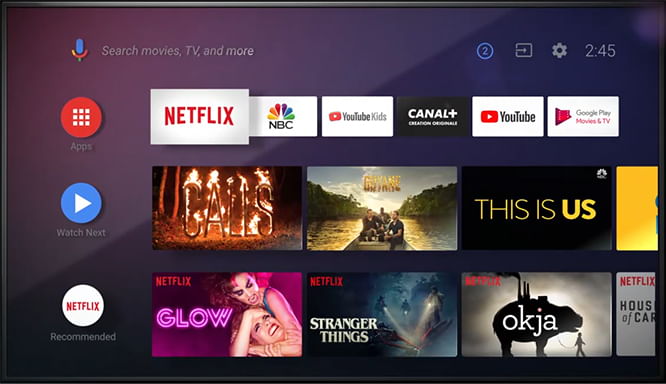The image depicts a TiVo-like user interface on a television screen, showcasing various internet services available for streaming TV shows directly on the TV. Prominently featured in the bottom right-hand corner is the Netflix app, accompanied by a "Recommended" tag for suggested content.

Above the Netflix app, there are two emoji icons – a blue emoji labeled "Watch Next" and a red emoji labeled "Apps". In the top left-hand corner, a search bar with a Google-styled microphone icon is present, indicating voice search functionality. The search bar displays the text "Search TV Movies, Search Movies TV and more," suggesting it is part of a Google-driven service.

The top right-hand corner includes icons for a clock, a settings gear, a broadcast button, and a button labeled "To." The main section of the interface presents a variety of viewing options including apps like Netflix, NBC, YouTube Kids, Canal+, YouTube, and Google Play. Among the highlighted TV shows and movies are titles such as "Calls," "This Is Us," "Glow," "Stranger Things," and "Okja," representing both NBC and Netflix content.

The background of the television app is predominantly purple, creating a cohesive and visually appealing interface.